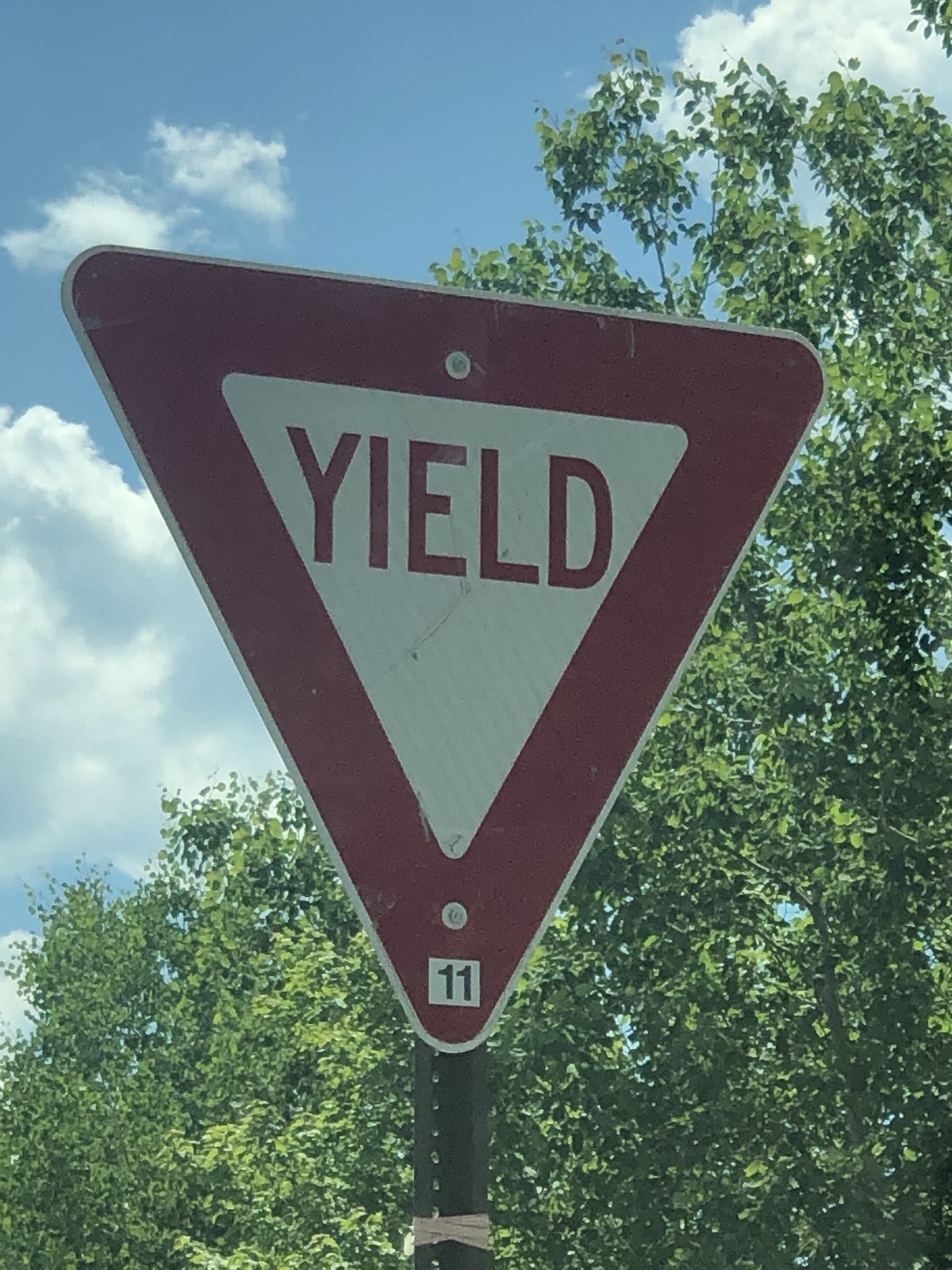The image depicts a large roadside traffic sign prominently featuring an inverted red triangle with a white triangular center. The word "Yield" is written in a slightly dull red color within this white triangle, indicating it is a traffic instruction sign. The sign is set against a vivid backdrop: on the right side of the image, there are lush green trees, while the left side showcases a bright blue sky dotted with fluffy white clouds. The scene is quite picturesque. Additionally, the traffic sign is numbered "11." The overall composition harmoniously combines the functional aspect of the sign with the natural beauty of the surroundings.